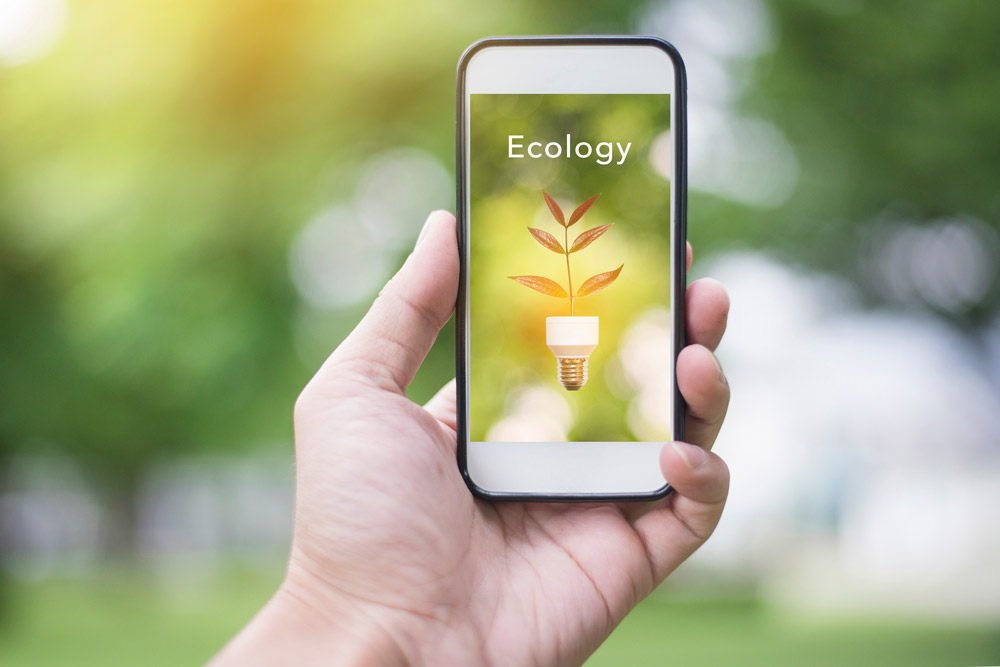In this color photograph, a person's left hand is prominently displayed, holding an older model iPhone towards the viewer. The focus is on the screen of the phone, which features the word "ecology" in white letters against a green backdrop. Below the text, there is an image of a light bulb with a plant emerging from its base, symbolizing a combination of nature and energy efficiency. The plant consists of brown leaves extending out of the light bulb's bottom part, designed to be screwed into a socket. The background of the photograph is deliberately blurred, featuring indiscernible green foliage, suggesting that the image was taken outdoors in a park or wooded area. No other objects or text are visible in the photograph, emphasizing the ecological theme displayed on the smartphone screen.